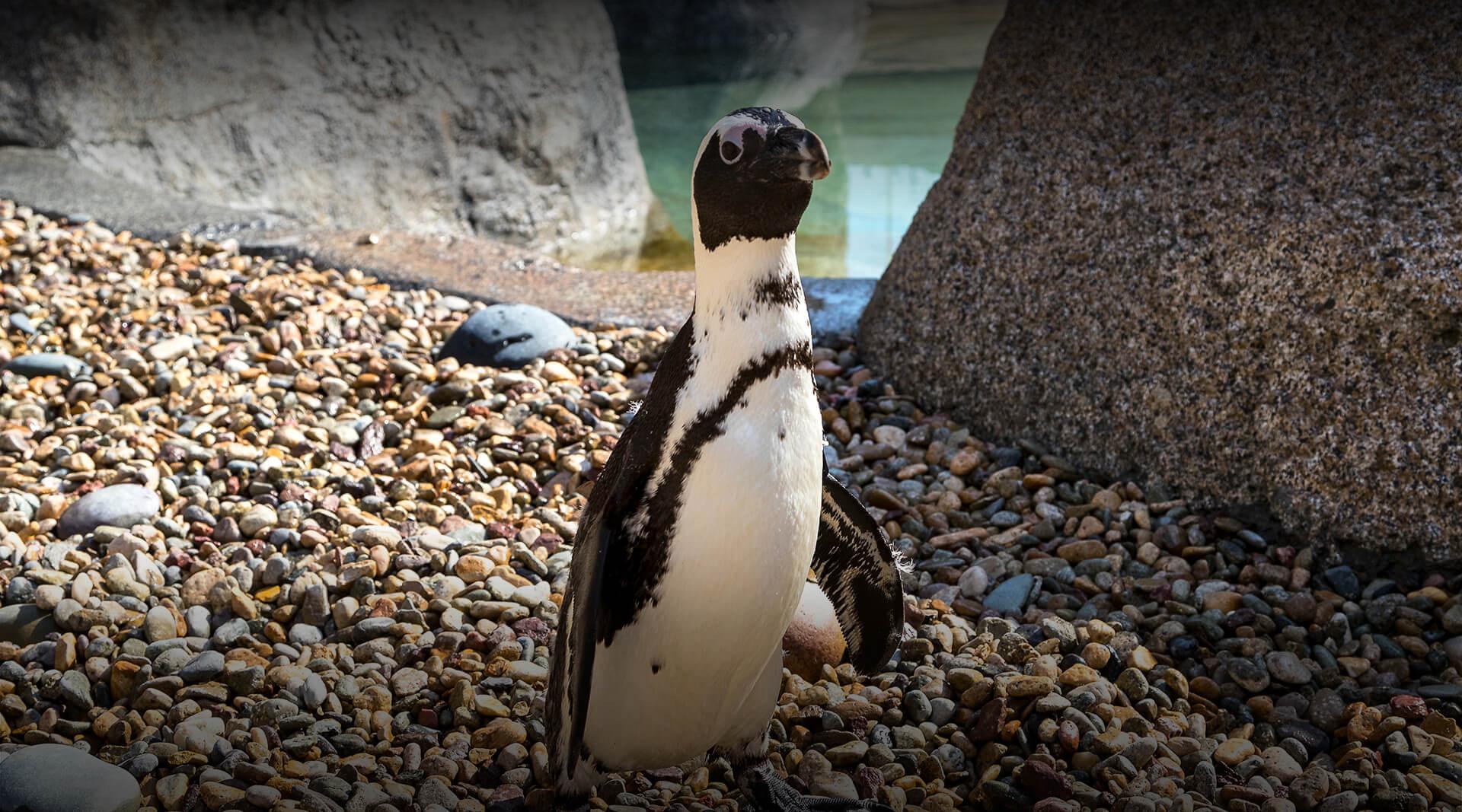The image showcases a close-up view of a small black and white penguin standing amidst an area densely covered with rocks. The rocks vary greatly in color, size, and shape, ranging from tiny pebbles to larger grey stones, creating a textured and diverse ground surface. Dominating the upper left and right corners of the image are two massive boulders, which frame the scene. Between these boulders runs a stone strip that leads down to a small body of water, resembling a pond. The penguin, appearing particularly diminutive against the vast array of rocks and boulders, adds a charming contrast to the rugged environment.